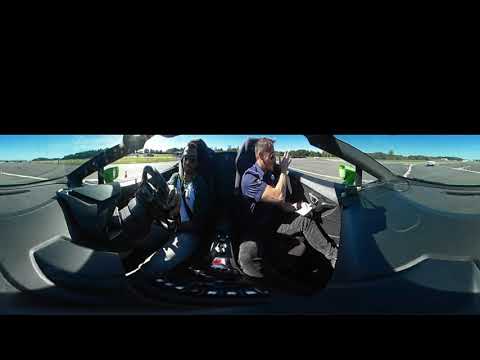The image captures the interior of a sporty, black or grey convertible car from a panoramic view, looking back at the driver and passenger. The driver's seat is on the left. The driver, seen with short black hair, a mustache, and facial hair around his chin, is wearing sunglasses, a black jacket over a white shirt, and blue jeans. He has his right hand on the steering wheel and his left arm resting by his body, with his seatbelt fastened. The interior features fancy, likely leather seats. The passenger to his right, dressed in a slightly more purplish blue t-shirt and black pants, has his hands raised, fingers spread, as if in mid-clap, and is also wearing sunglasses. The scene outside the open roof reveals a clear blue sky with the sun shining, an asphalt area that resembles a raceway or an airport takeoff zone, and a backdrop of trees and grass. Additionally, there's a light green car mirror and a single white car visible on the road behind them.